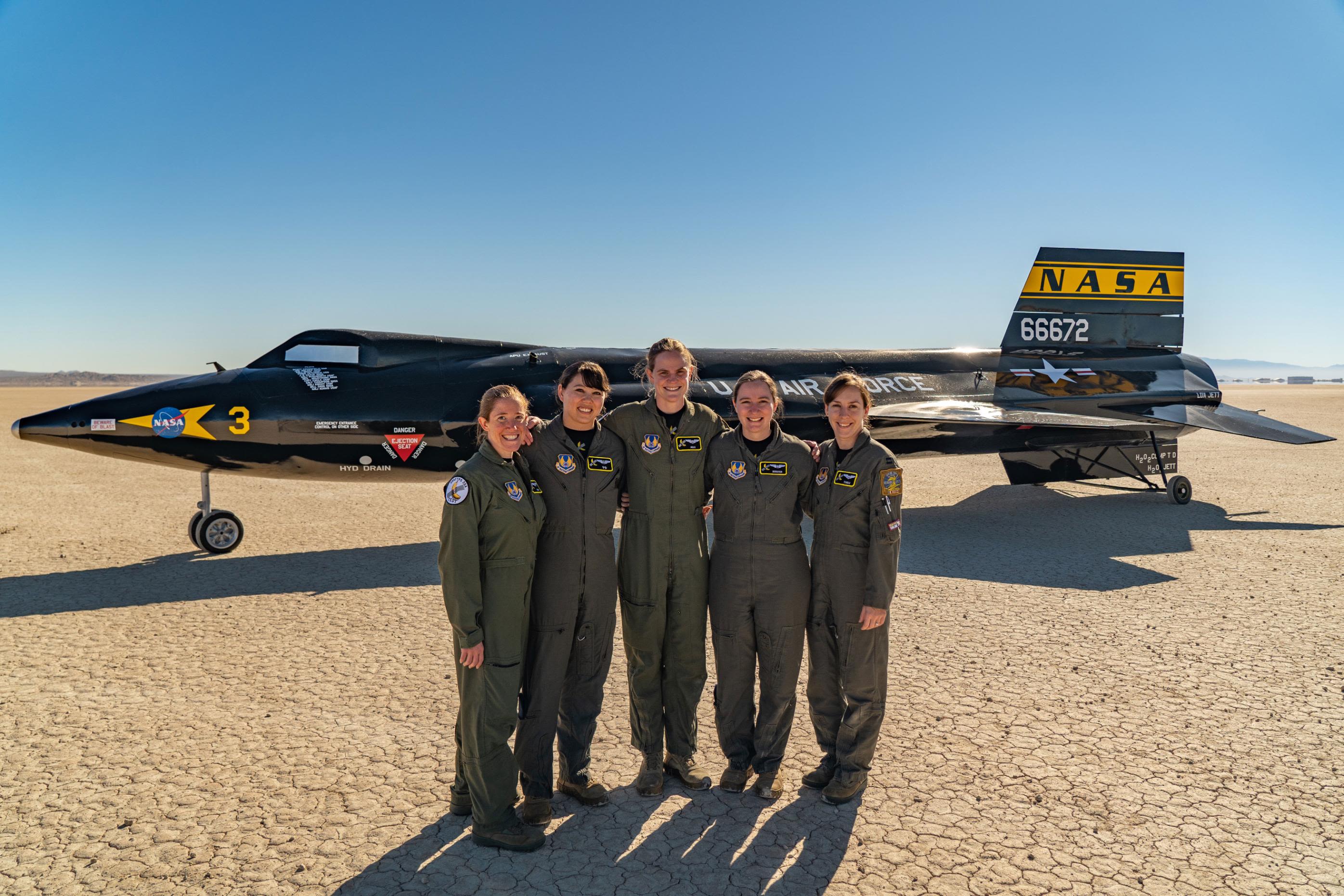The photograph captures a vibrant scene featuring five women standing shoulder to shoulder, all smiling warmly in military green flight jumpsuits adorned with various patches on their shoulders and chests. They pose in front of a sleek, black U.S. Air Force jet with the number "66672" and a star emblazoned beneath it. "NASA" is prominently displayed on the tail, and "US Air Force" is written on the body of the jet. The clear blue sky overhead transitions to a faint white at the horizon, where distant hills are visible. The setting appears to be an arid desert with cracked, sandy-colored ground stretching flat and wide under the bright sun, casting their shadows towards the viewer.